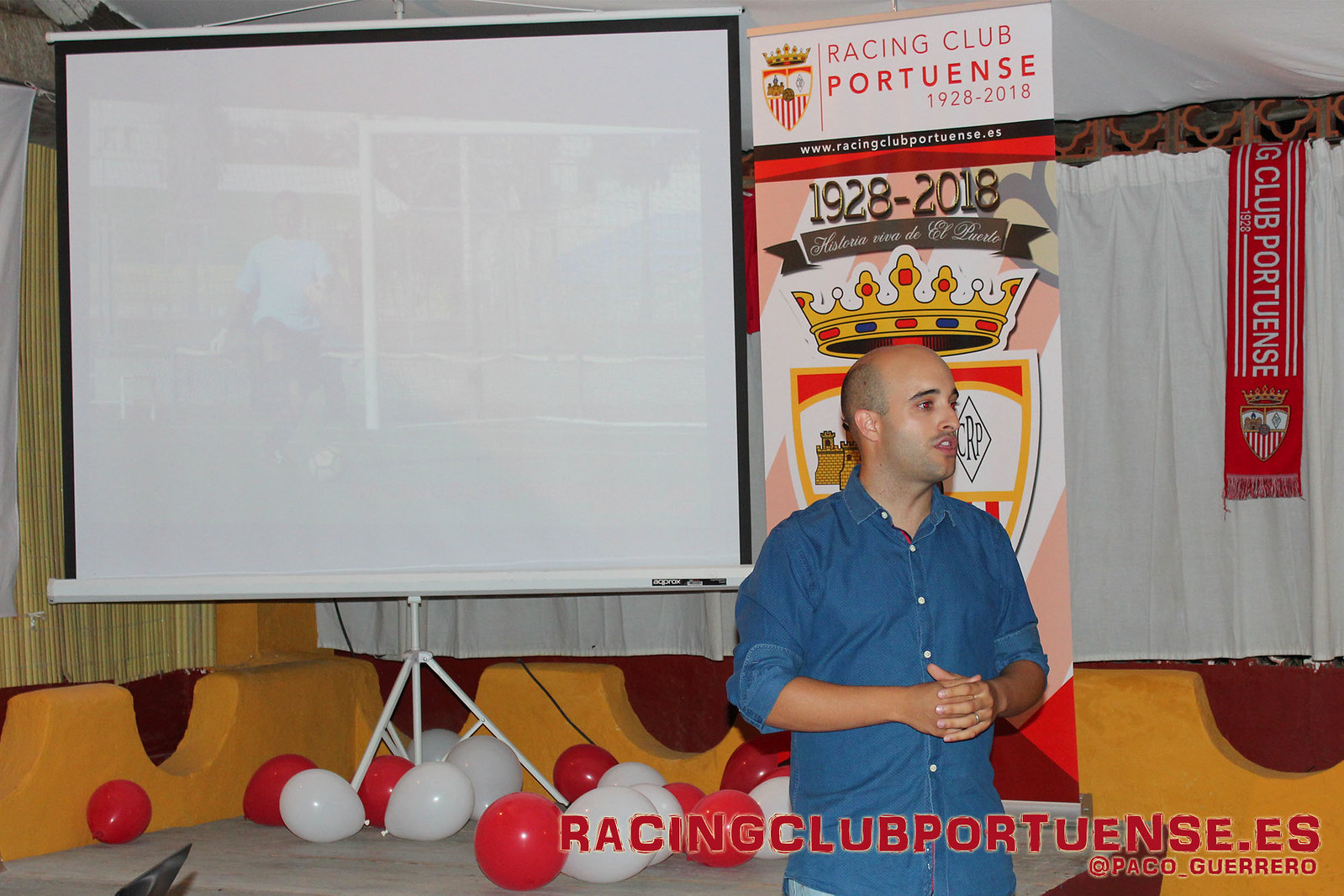In this detailed indoor image, a man stands in front of a white projector screen, giving a presentation. He wears a blue shirt with rolled-up sleeves and light blue jeans. His head is almost fully shaved, revealing a receding hairline. Behind him is a large banner that reads "Racing Club Portuense 1928-2018" in bold lettering. The banner, predominantly red, yellow, and white, features a prominent crown and a partially obscured shield emblem, possibly depicting a castle. Below the projector screen, a collection of white and red balloons is scattered on the ground. To his right, another banner displays "Club Portuense" with the same crown and shield insignia. On the bottom of the image, the URL "racingclubportuense.es @Paco_Guerrero" is visible. The projector screen faintly shows an image of someone playing soccer, adding an active element to the otherwise static scene.